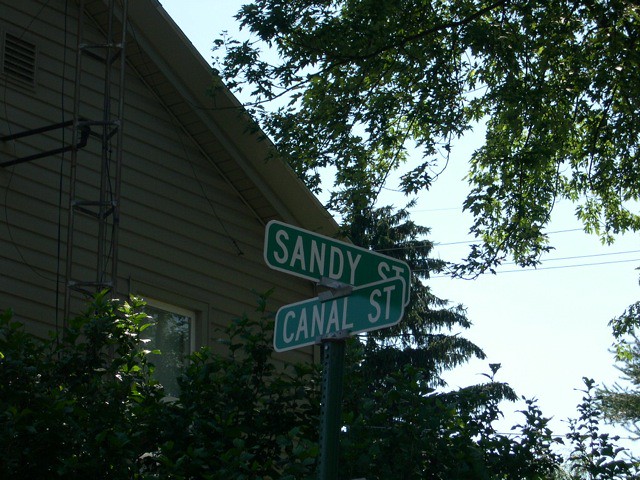This detailed photograph captures an intersection marked by two street signs, prominently placed on top of a green metal signpost. The top sign reads "Sandy Street," facing slightly to the right, while the bottom sign reads "Canal Street," slightly facing to the left, both clearly legible from the camera's perspective. The scene is bathed in daylight, with sunlight enhancing the visibility and details of the surroundings.

In the background, a gray house with horizontal wooden paneling occupies the left half of the image. The house features an angled roof, a single window, and some metal scaffolding in front of it. Below the window, low-growing hedge-type shrubs add a touch of greenery. To the right of the house stands a pine tree, and in the upper right corner of the photograph, a large deciduous tree extends its branches downward, contributing to the serene and natural backdrop of the image.

Above it all, a clear, light blue sky with hints of white adds to the overall clarity and bright atmosphere of the photograph, creating a pleasing contrast with the green foliage and the muted tones of the house.